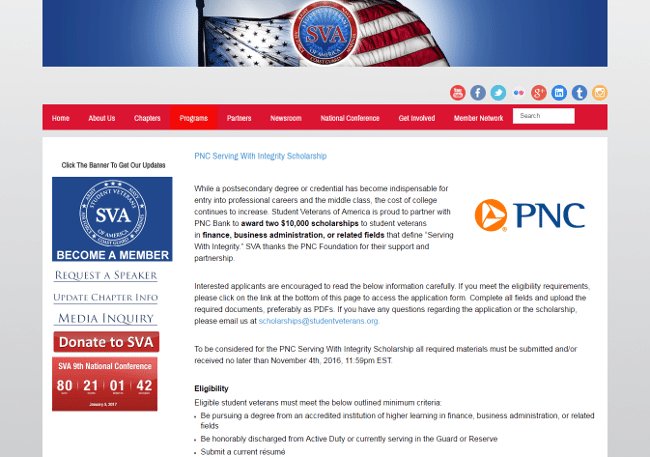The image is a screen capture of the SVA (Student Veterans of America) website, specifically on the "Programs" tab, detailing the "PNC Serving with Integrity Scholarship." At the very top of the screen, there is a banner featuring an American flag on a blue background, with the flag partially visible. Centered on this banner is a seal displaying the acronym "SVA" in red font, set against a blue backdrop with a red border.

Just below this banner, there's a gray interim section that serves as the background of the web page. Within this section are icons linking to various social media platforms, including YouTube, Facebook, Twitter, an icon with a blue and green circle likely representing an additional social network, Google Plus, LinkedIn, Tumblr, and Instagram.

Further down, a navigation banner features buttons labeled Home, About Us, Chapters, Programs, Partners, Newsroom, National Conference, Get Involved, Member Network, accompanied by a white search box.

To the right of this banner, a PNC logo is displayed, characterized by a triangular shape within a circle. The main headline, "PNC Serving with Integrity Scholarships," is prominently featured at the top of the page. On the left-hand side, another SVA logo is visible, this time in white text against a blue background, accompanied by the invitation to "Become a Member."

Below this logo, several additional options are listed: "Request a Speaker," "Update Chapter Info," and "Media Inquiry."